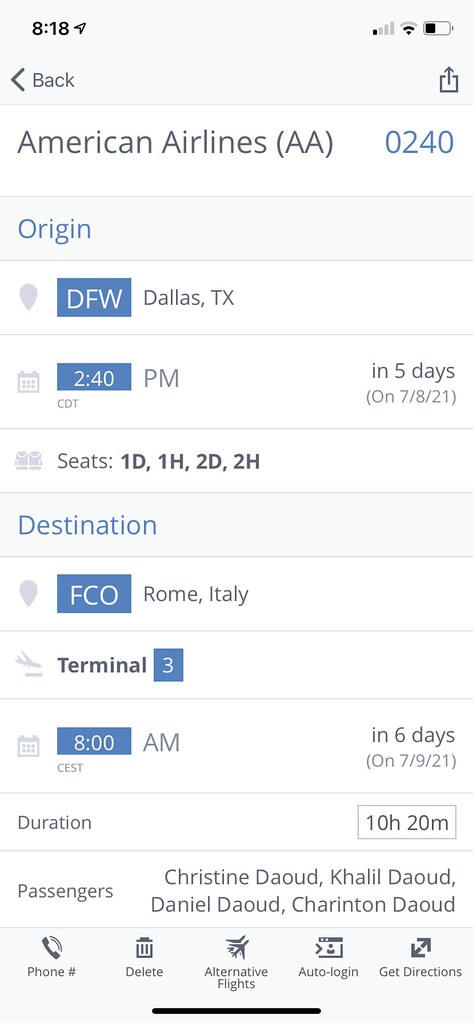**Detailed Flight Confirmation Information Screenshot - American Airlines**

This screenshot is a mobile view of the flight confirmation details for an American Airlines flight.

1. **Screen Status Bar**:
   - **Time**: Displayed on the upper left is "8:18".
   - **Compass Navigation Arrow**: Points towards the northeast.
   - **Cellular Signal**: One of four bars is active, with the remaining three grayed out.
   - **Wi-Fi Strength**: One of two bars is active.
   - **Battery Level**: Indicated at 40%, shown through a black icon with a white battery symbol.

2. **Navigation and Menu Options**:
   - **Back Button**: Displayed as a black text with a bracket arrow facing to the left.
   - **Upload Button**: Positioned on the right.

3. **Flight Information**:
   - **Airline**: American Airlines (AA).
   - **Flight Number**: 0240 (highlighted in blue).

4. **Origin Details**:
   - **Row Background**: Light gray.
   - **Icon**: A gray location marker resembling a balloon.
   - **Airport Code**: DFW (in a blue box).
   - **Location**: Dallas, TX (in gray text).

5. **Departure Details**:
   - **Calendar Icon**: Light gray.
   - **Time**: 2:40 PM (displayed in a blue box with white text and "PM" in gray).
   - **Time Zone**: CDT (Central Daylight Time).
   - **Days Remaining**: "In five days", with the date beneath it (7-8-21).

6. **Passenger Seats**: 
   - **Seats Assigned**: 1D, 1H, 2D, and 2H.

7. **Destination Details**:
   - **Row Background**: Light gray to highlight.
   - **Icon**: Same gray location symbol.
   - **Airport Code**: FCO (in a blue box).
   - **Location**: Rome, Italy.
   - **Terminal**: Terminal 3 (with "3" in a blue box).

8. **Arrival Details**:
   - **Arrival Time**: 8:00 AM CEST (Central European Summer Time).
   - **Days Remaining**: "In six days", with the date beneath it (7-9-21).

9. **Flight Duration**:
   - **Duration**: 10 hours and 20 minutes (enclosed in a gray-outlined box).

10. **Passenger Information**:
     - **Passengers**: Christine Dayoud, Khalil Dayoud, Daniel Dayoud, Cheryantan Dayoud.

11. **Footer Menu Options**:
    - **Phone Number**: With a calling icon.
    - **Delete**: With a trash can icon.
    - **Alternative Flights**: Represented by two overlapping airplane icons.
    - **Auto-login**: Shown with a web page icon and a right bracket.
    - **Get Directions**: Displayed with intersecting arrows pointing to the lower left and upper right.

12. **Dividing Line**:
    - **Separator**: A black horizontal line at the bottom middle section of the screenshot.

This precise and detailed information provides a clear view of the flight's logistical details and associated passenger data, punctuated by user interface elements for ease of navigation and options management.